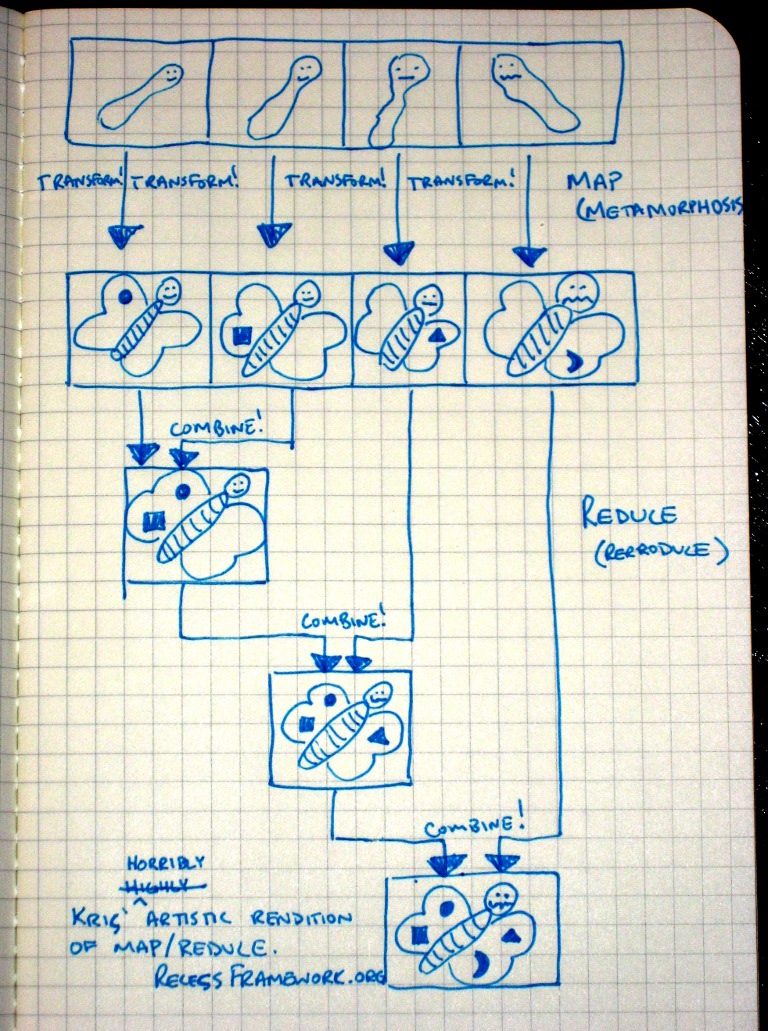This photograph captures a page from a student's workbook, most likely designed for educational purposes. The page features square, graph-style paper, commonly used for diagramming. Centered on the page is a detailed flowchart explaining the metamorphosis of a caterpillar into a butterfly. 

At the top of the flowchart are four boxes, each containing a thin, blob-like shape with a smiley face, varying slightly in size, growing progressively larger from left to right. These shapes represent the stages of caterpillar growth. Arrows guide the viewer's eye downward from these boxes to a second row of four boxes. Inside these, there are various butterfly shapes, each with uniquely shaped wings.

Further arrows lead from these butterfly boxes to a third row, which consolidates into three boxes. These final boxes discuss the combination of different species to create butterflies with two, three, or four distinct wing shapes. The flowchart provides a clear, step-by-step visual description of the transformation process from caterpillar to butterfly.